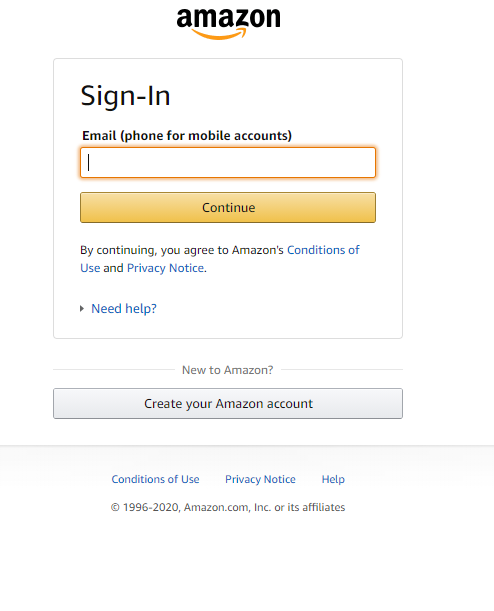The image is a screenshot from the Amazon login page. The background is white, and at the top center of the page is the Amazon logo, featuring black text with a yellowish-orange arrow that extends from the letter "A" to the letter "Z," symbolizing the company's wide range of products.

Directly beneath the logo is a rectangular box titled "Sign-In" positioned in the upper left corner. Below this heading, there's a prompt in black text that reads, "Email or mobile phone number," indicating where users should enter their login credentials. There is a blank input field waiting for an email address or phone number.

Under the input field is a yellowish-orange button labeled "Continue," which users click after entering their information. Further down, there's a line of text stating, "By continuing, you agree to Amazon's Conditions of Use and Privacy Notice."

At the bottom of the box, there is a "Need help?" button followed by a link that says, "New to Amazon? Create your Amazon account," inviting new users to register.